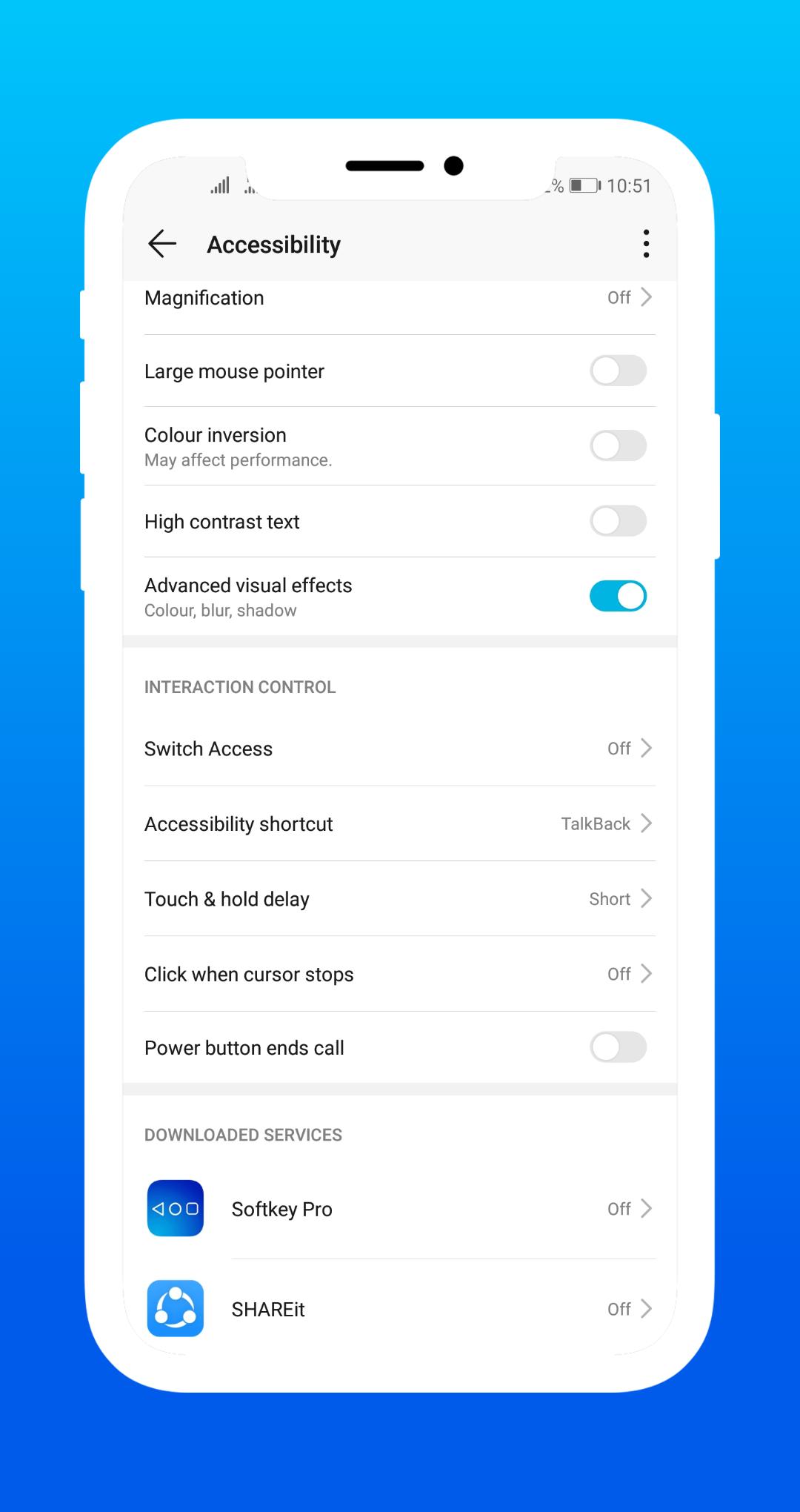This image is a detailed screenshot of the "Accessibility" settings on an iPhone. The screenshot is bordered by a light blue frame, with a centered white rectangular screen that has rounded corners. At the top of the screen, there is a status bar that includes a short black line with a little black circle next to it, indicative of signal strength, and a small percentage sign displaying the battery level, which is less than half full, along with the current time, "10:51." On the left side of the status bar, there are internet access bars and some other icon, followed by what appears to be a search bar below that, labelled "Accessibility," with an arrow pointing left and three dots on the right.

The main settings page begins with a section labelled "Magnification" on the left and an "Off" status with an accompanying arrow on the right. This is followed by lines separating each setting. The next options include: "Large Mouse Pointer," "Color Inversion," which has a note indicating that it "may alter performance," "High Contrast Text," and an option for "Advanced Visual Effects," which is toggled on. Additional settings listed include: "Color," "Blur," and "Shadow."

Further down, a darker line separates the previous settings from the "Interaction Control" section. This section includes options such as "Switch Access," "Accessibility Shortcut," "Touch and Hold Delay," "Click When Cursor Stops," and "Power Button Ends Call."

Below these settings, there is another section titled "Downloaded Services," featuring two blue icons: "SoftKey Pro" and "SHAREit" indicated by an image of three circular dots arranged in a circular arrow pattern. To the right of the screen, there is a series of toggle buttons to switch these settings on or off, with the "Advanced Visual Effects" option being the only one toggled on.